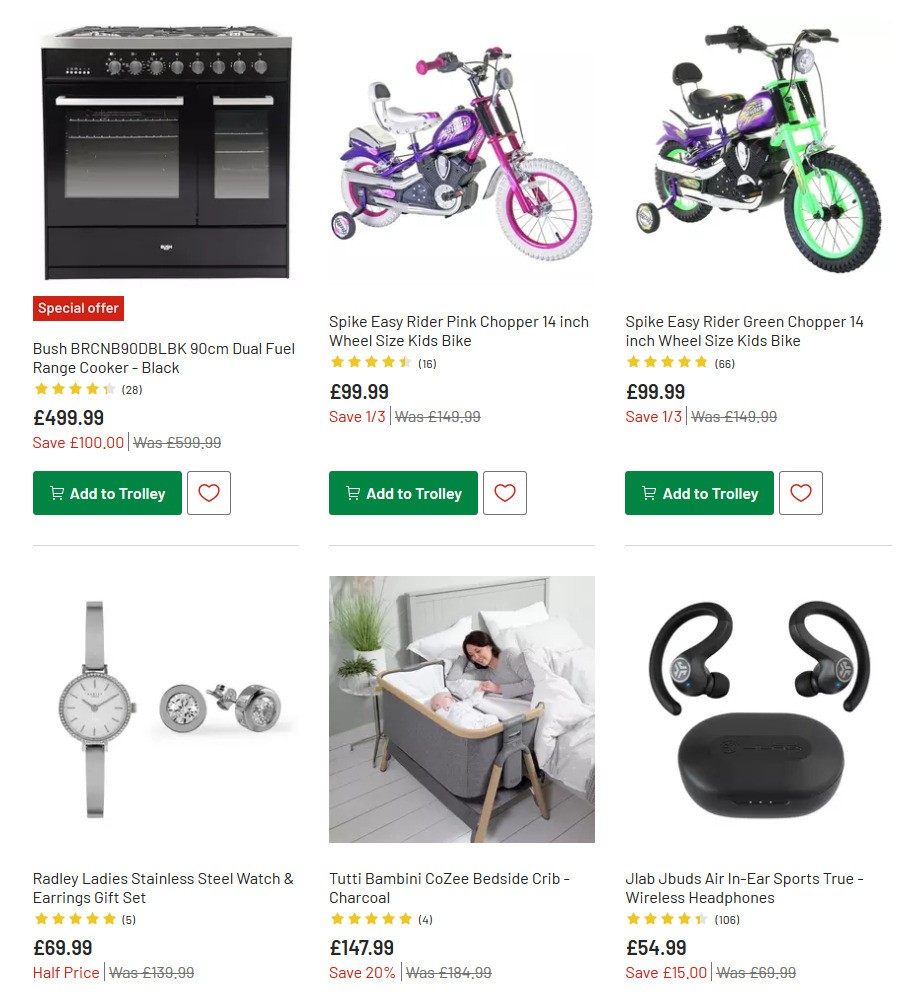This image portrays a webpage, likely from the Amazon UK website, showcasing a variety of goods and services. Featured prominently are six distinct items. The first is a black dual fuel range cooker priced at £499. Next is a children's bike, labeled "Spike Easy Rider Pink Chopper," equipped with training wheels and costing £100. Alongside it, there is another bike, a "Green Chopper," also priced at £100, characterized by its unique design.

Additionally, a ladies' stainless steel watch and earring gift set is displayed for £70. The page also features a bedside crib depicted with a mother resting in bed beside her newborn, available for £147 with a 20% discount. Lastly, the JLab JBuds Air Sports True wireless headphones are listed at £5,499, with an additional £15 savings offered.

The webpage includes an "Add to trolley" option, equivalent to "add to cart," indicating that these items are ready for purchase. The overall layout suggests a typical online shopping experience, with various products available for browsing and buying from the UK-based platform.